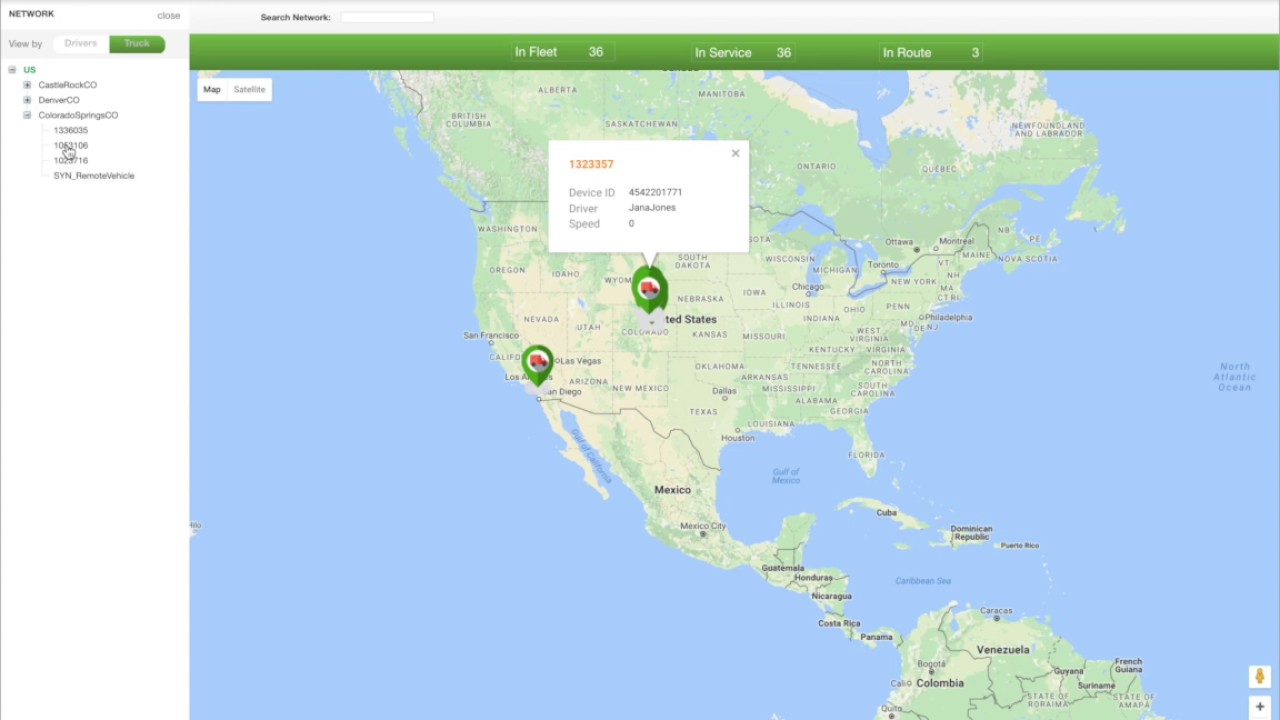This image depicts a detailed digital interface page, primarily showcasing a map of North America with adjacent regions and a tracking system.

At the very top of the page, a one-inch white strip spans the width of the interface. From the left, a two-inch wide white column extends top to bottom, acting as a sidebar. The rest of the page is dominated by a large map.

In the top-left corner of the page, "NETWORK" is displayed in bold, black, all-capital letters. Approximately an inch to the right is the word "Closed" in smaller black lettering, followed by "Search Network" and a search bar beneath it. Below "NETWORK," there is an option to view by a category featuring a white tab labeled "Drivers" in black text and a green tab labeled "Truck." Under the green tab, it reads "US."

Adjacent to this section are headings with location names: "Castle Rock CEO," "Denver CEO," and "Colorado Springs CEO," followed by some numeric device ID details, although their specific purpose is unclear.

The map itself is bordered in green with white text stating, "In Fleet 36," "In Service 36," and "In Route 3." In the top-left corner of the map, a white and black rectangular area provides the options for "Map" and a divided subsection labeled "Satellite."

The central map portrays North America in detail, with a portion of South America visible toward the bottom-right corner. The Atlantic and Pacific Oceans are shown in blue. Canada is predominantly shaded in green, except for its northeastern region. Most of the United States is depicted in a whitish hue with some green areas, similar to Mexico and parts of South America. Notably, there are green pins marking locations in Colorado and Los Angeles.

This comprehensive page effectively combines map visualizations with logistical data, offering a clear display of fleet and route information.